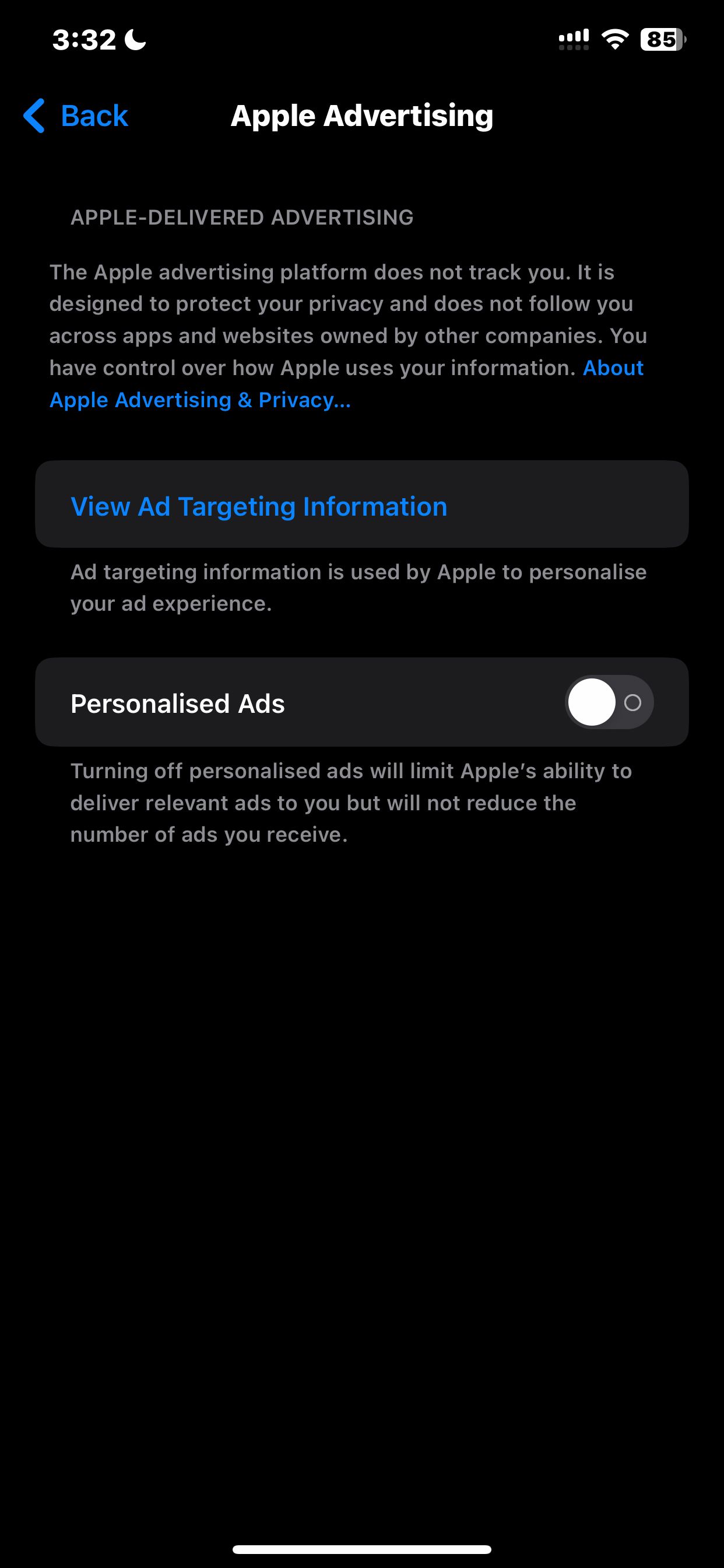The image depicts a phone screen with a black background and white text. At the top left corner, there is a timestamp showing "3:32" with a crescent moon icon to indicate night mode. To the right of the timestamp, the Wi-Fi signal icon and a battery icon display a battery level of 85%. 

Immediately below in blue, there is a back arrow icon next to the word "Back" followed by the title "Apple Advertising" in white font centered on the screen. Below it, in a lighter gray font, the text reads, "Apple-delivered advertising."

Continuing down, the next section states, "The Apple Advertising Platform does not track you; it is designed to protect your privacy and does not follow you across apps and websites owned by other companies. You have control over how apps use your information." Following this in blue font is a link labeled "About Apple Advertising and Privacy."

Encased within a gray rectangular box, there is a blue text link that reads "View Ad Targeting Information." Outside of this gray box, the black font continues with the text, "Targeting information is used by Apple to personalize your ad experience."

To the right side, inside a gray circle, there is white text that says "Personalized Ads." Next to it on the right is a large white circle followed by a gray circle with a faint whitish outline. Below this, more gray font states, "Turning off personalized ads limits Apple's ability to deliver relevant ads to you but will not reduce the number of ads you receive."

At the bottom of the screen, there is a thick white line running horizontally across the middle, likely used to provide navigational options or to separate sections within the interface.